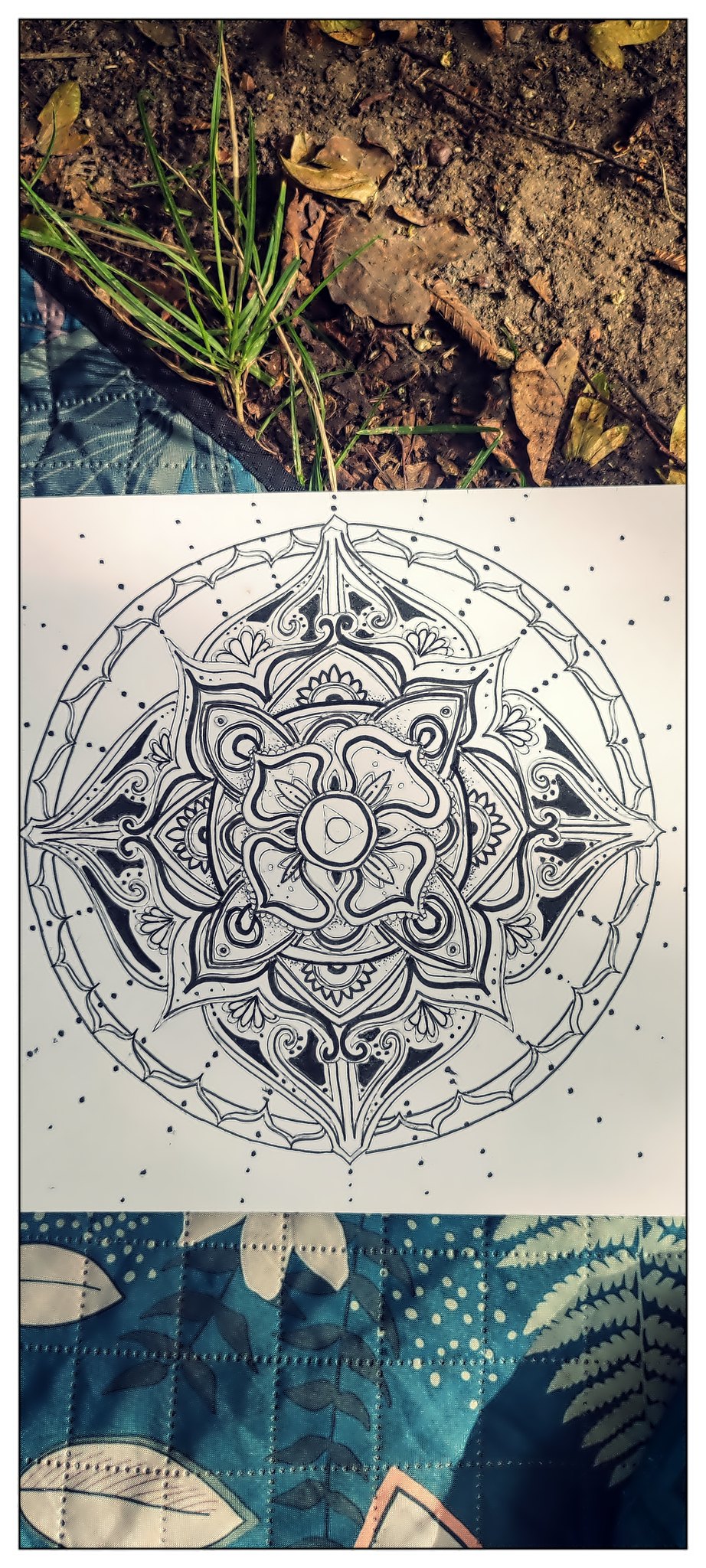The image captures an outdoor nature setting, possibly from a picnic, hiking excursion, or camping trip. A blanket, blue with white leaves, is spread out on the dirt, partially reaching onto a small patch of green grass. On the blanket, extending onto the ground, lies a white sheet of paper featuring an intricate black and white drawing. The artwork showcases a detailed, ornate mandala design. The pattern begins at the center with a flower, expanding outward in layers that alternate between various floral forms. The petals increase in size with each layer, eventually forming a diamond shape surrounded by a larger encompassing circle adorned with dots. The scene suggests that someone ventured into nature to creatively express themselves through art, beautifully blending the serene environment with their elaborate drawing.